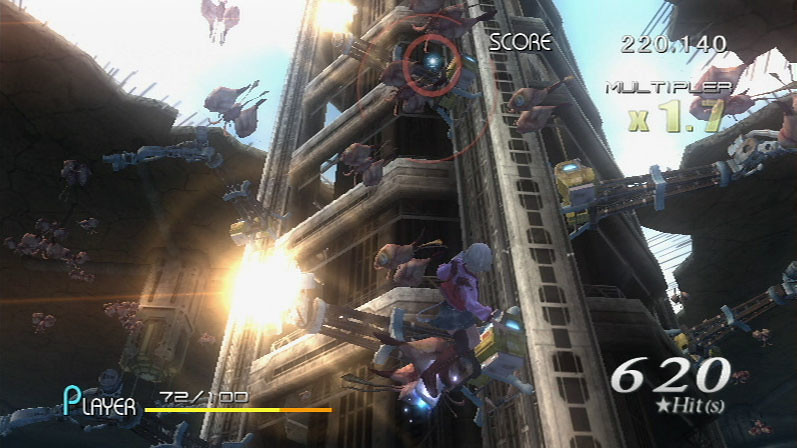This image is a detailed screenshot from a sophisticated, modern video game, likely a multiplayer FPS shooter. Dominating the center of the scene is a large, multi-story grey tower that extends off the top of the screen, giving off a brutalist architecture vibe. The foreground features multiple heavily armored action figures, some equipped with Gatling guns, actively shooting. Notably, there's a pronounced muzzle flash from one of these guns near the center, directed toward the tower. Above, various winged creatures or small spacecraft are seen flying against a blue and white sky, adding to the intense atmosphere.

On the bottom left corner, there is a life bar reading "player" in white text with a blue "P," showing "72/100" over a yellow-to-orange gradient, indicating the player's remaining life force. The bottom right corner displays "620" followed by "star hits" with an "S" in parentheses, while the upper right corner reads "220,140" alongside a "multiplier X 1.7" in yellow text. Additional visual effects like light lens flares contribute to the overall dynamic and high-energy visual experience of the game.